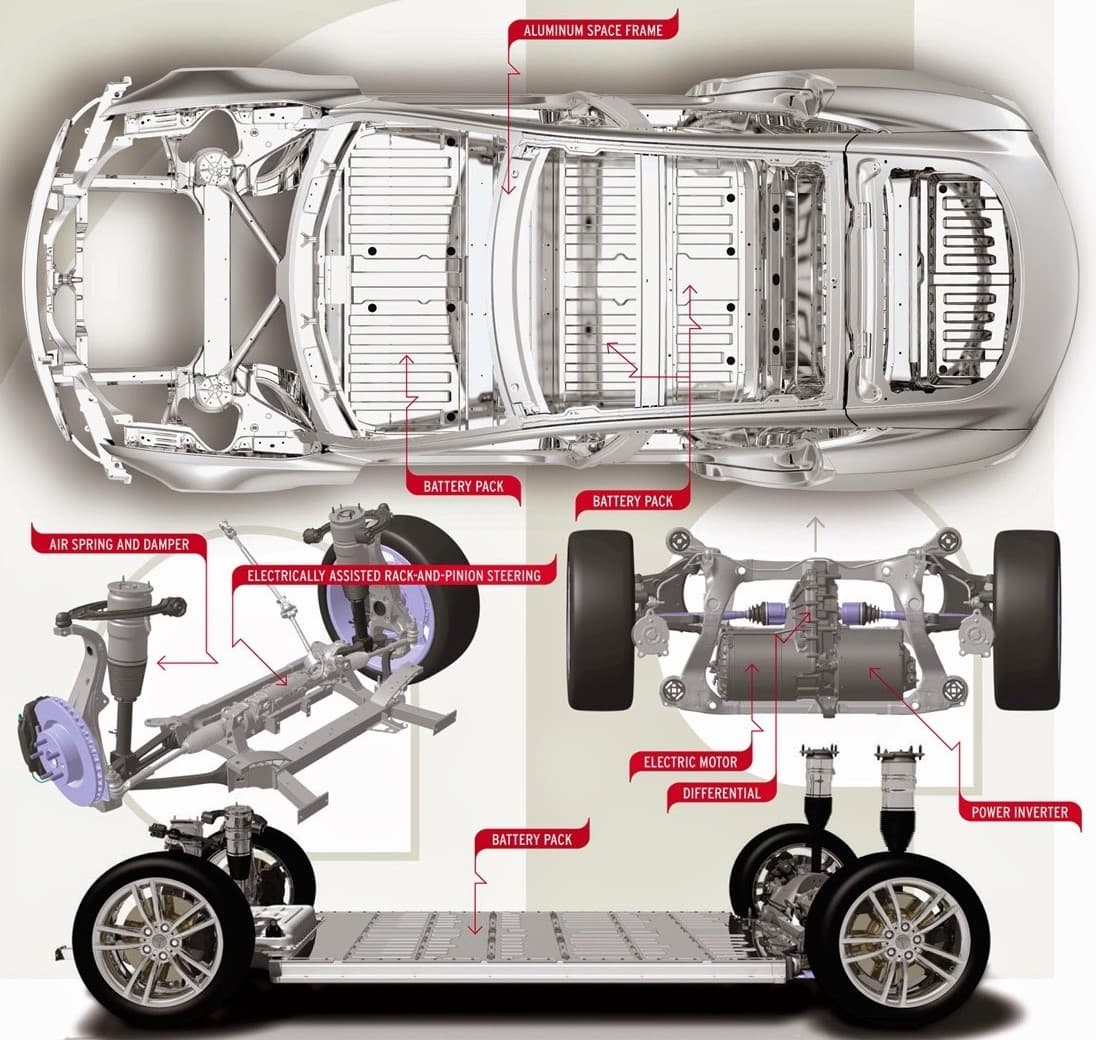The image is an intricate rendering of an electric vehicle, composed of detailed, labeled diagrams, showcasing various key components in a deconstructed view. Dominating the top section is an overhead view of the aluminum space frame, visually separated from the rest of the car to highlight its structure. Red arrows with white text labels point to essential areas, such as the "aluminum space frame."

Below, the diagram elaborates on the wheel assembly, exhibiting specific parts like the air springs, dampers, and the electrically assisted rack and pinion steering. Black tires and suspension components are meticulously detailed, emphasizing their standalone structure when detached from the car.

The bottom part of the image highlights the car's battery pack and its configuration when integrated with the wheels and the framing. Labels point out the "battery pack," "electric motor," "differential," and "power inverter," with red flags and text bringing attention to each component. The primary colors used in the rendering are gray and white, with the textual annotations and arrows in red for emphasis.

Overall, the image serves as a comprehensive dissection of the electric vehicle, providing a thorough visual understanding of its frame, wheel assembly, and power components.